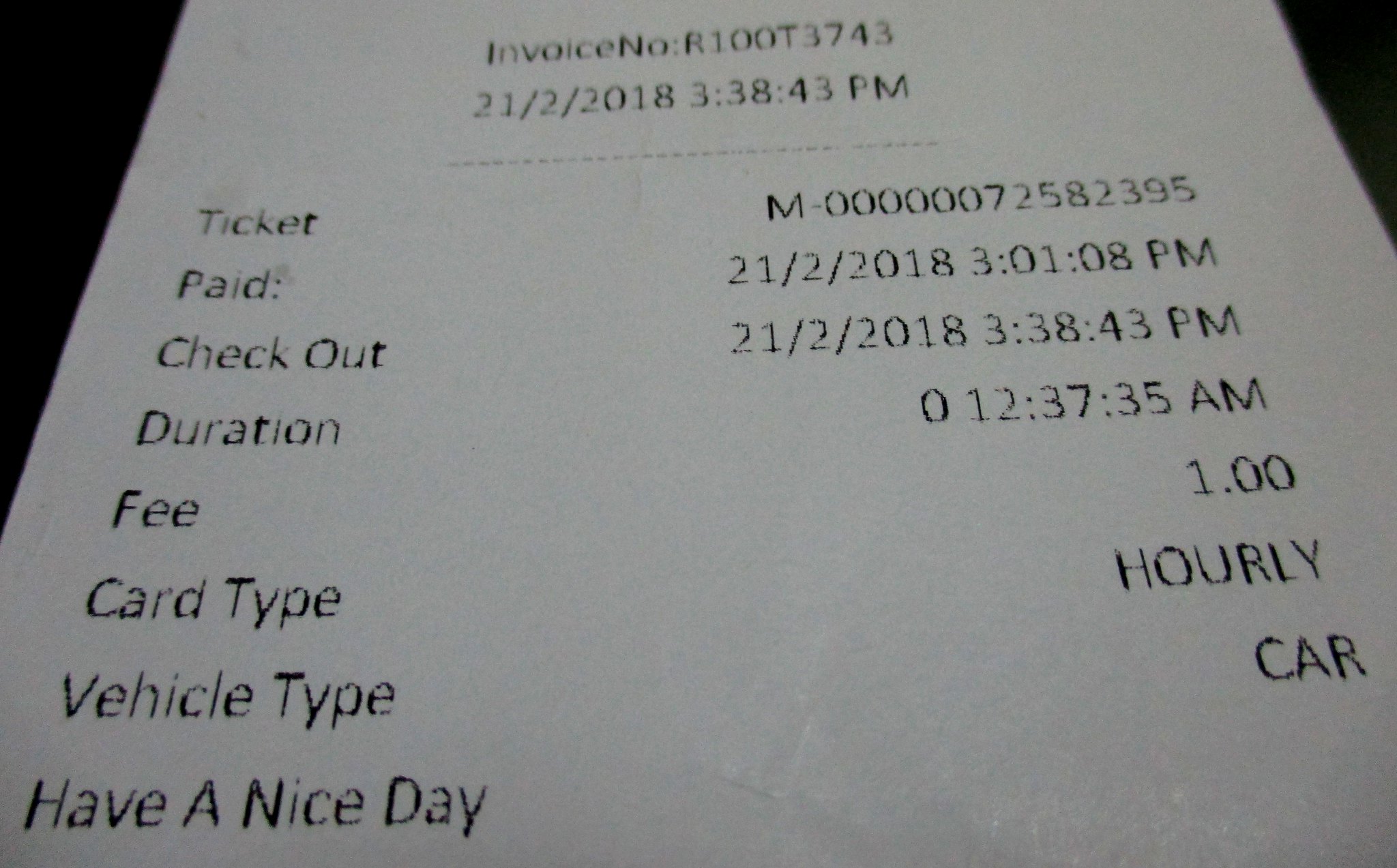This image is a close-up photograph of a parking receipt against a white background with simple black text. The receipt is slightly oriented away from us at the top, bringing the bottom part into clear view in the foreground, and there is some black visible behind the receipt on the upper left and upper right. 

At the very top, the invoice number "R100T3743" is prominently displayed, followed by the date "February 21, 2018," and the exact time "3:38:43 PM." Beneath this, on the left side, several details are listed in two columns: 
- Ticket: M00000072582395
- Paid Time: 3:01 PM
- Checkout Time: 3:38 PM
- Duration: 12 minutes 37 seconds
- Fee: $1
- Card Type: 
- Vehicle Type: Car

The right side column matches the left in structure, showing the same categories justifying the details, such as payment information and timings. Near the bottom left of the receipt, there's a friendly note saying "Have a Nice Day."